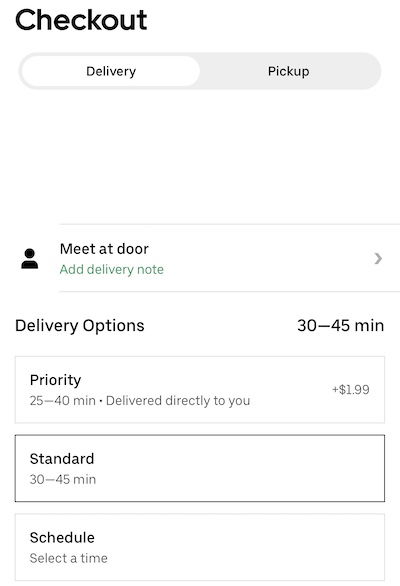In the image, the overall background is white. At the very top, in black text, it reads "Check Out." Directly below this line of text is an oval that is divided into two sections: the left half is white with black text that says "Delivery," and the right half is gray with black text that says "Pick Up." Below this element is a thin gray line, beneath which, in bold black text, it states "Meet at Door." Further down, the text "Add Delivery Note" is displayed in gray.

Additionally, there is a small icon of a person beneath these instructions. Under this icon, "Delivery Options: 30 to 45 minutes" is written in bold black text. Below this section are three rectangular options, each having a white background. The top rectangle has a light gray thin outline and features black text that reads "Priority." Below this, in light gray text, it details "25 to 40 min, delivered directly to you + $1.99." The middle rectangle is outlined in a darker gray with the text "Standard" and "30 to 45 minutes" written in black. The bottom rectangle is outlined in light gray and reads "Schedule: select a time" in black text.